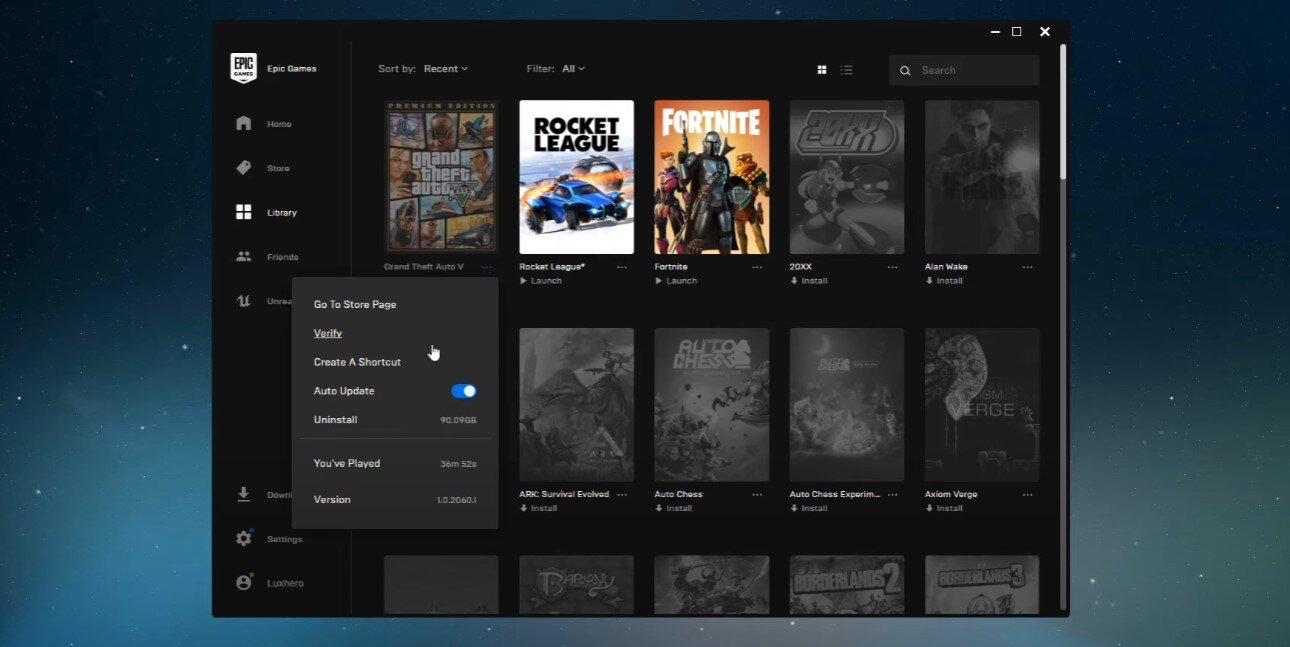This detailed image is a screenshot from the Epic Games launcher. Prominently, at the top left of the central app window, the Epic Games logo is displayed. The logo has a shield-like shape with the word "Epic" at the top and "Games" below it. 

The outer edges of the image are colored with a bluish tint, evoking a spacelike atmosphere dotted with numerous white stars, creating a galactic background.

Within the Epic Games app window, the left sidebar showcases several categories, each accompanied by an icon. These categories include:
- **Home** with a house icon
- **Store** with a shopping tag icon
- **Library** with a grid of four squares
- **Friends** with a two-person icon
- **Unreal** with a stylized "U" icon

Below these main categories, an additional section features:
- **Downloads**
- **Settings**
- The username of the person's account

In the central section of the image, there are three rows of game thumbnails, each row containing five games. Notably, the top left three games are highlighted: 
- **Grand Theft Auto V**
- **Rocket League**
- **Fortnite**

This detailed arrangement provides a comprehensive view of both the structure and content of the Epic Games launcher interface.